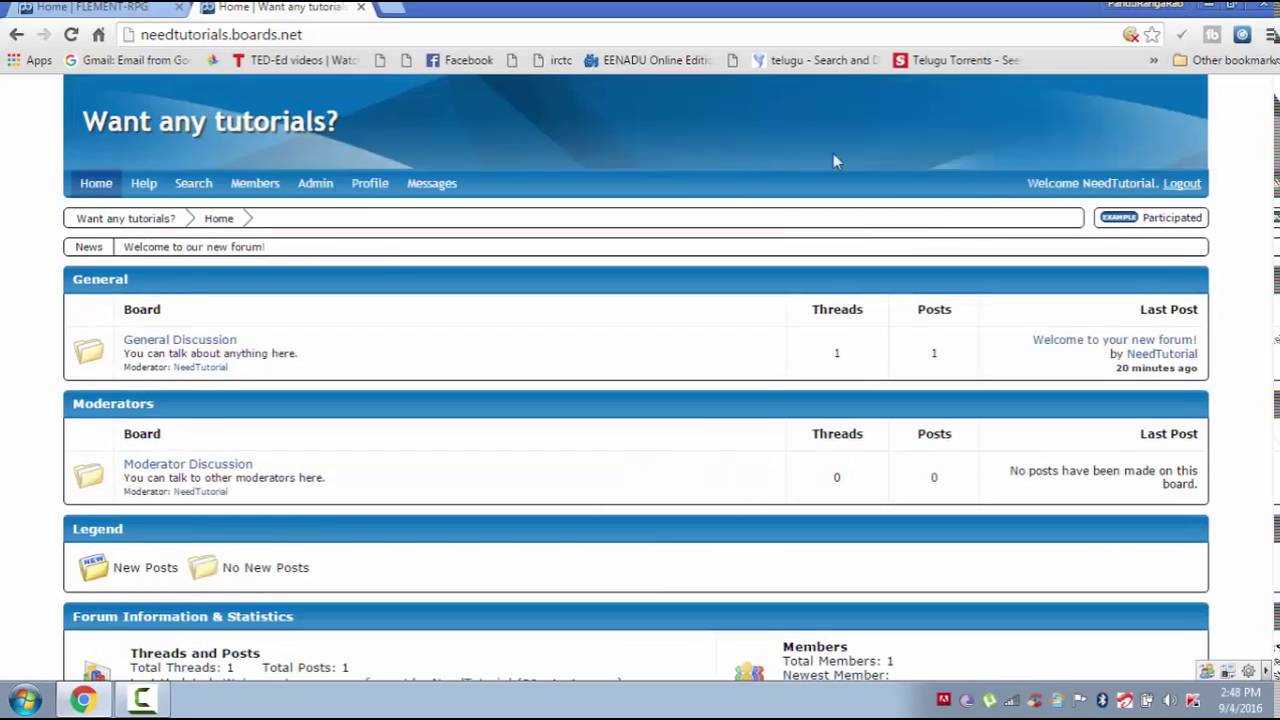This screenshot captures a partial view of an old Windows interface, specifically from within the Google Chrome browser. The top part of the image is slightly cut off, but it's clear that two tabs are open. The active tab is the rightmost one with the URL bar displaying "neatutorials.boards.net." Standard browser navigational icons, such as the back button, are present. Beneath the address bar are a series of bookmarked items including "Apps," "Gmail," "TED," and "Facebook," alongside several document icons without labels. Additional bookmarks include "eenaduonline," "Telugu search," and "Telugu torrents," with "Other Bookmarks" listed on the right side.

The primary content of the page features a blue header reading "Want any tutorials?" Below this header, typical navigational links, likely including "Home," are slightly obscured. The main area is divided into sections with black and blue-outlined boxes containing folder icons and possible table elements. 

The first section, labeled "General" in a blue header, includes the board "General Discussion" with columns for "Threads," "Posts," and "Last Post." Details within this section indicate one thread and one post, though the last post is unreadable. The next section, titled "Moderators," follows a similar layout but indicates zero threads and posts.

A blue box labeled "Legend" explains forum features with icons for "New Posts" and "No New Posts." Below this, another section likely labeled "Forum Information and Statistics" is partially cut off, rendering the text unreadable.

Finally, the image includes a taskbar at the bottom, characteristic of a Windows 10 environment, displaying the Chrome icon among other application icons.